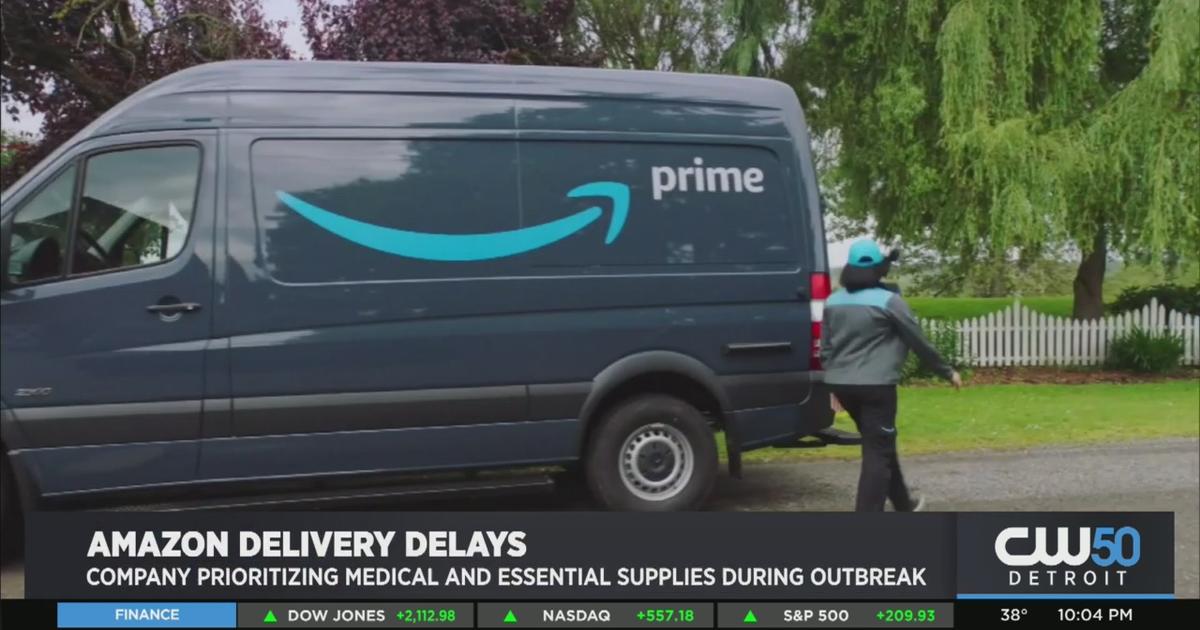The screenshot from Adford Prime depicts a serene residential neighborhood, featuring a picturesque grassy yard enclosed by a charming white picket fence with varying heights. The well-maintained yard includes lush bushes and trees, adding to the idyllic scenery. Parked on the road in front is an Amazon Prime delivery van, prominently displaying the distinctive blue "Prime" logo. In the foreground, a delivery person is present, dressed in black slacks and black tennis shoes with white soles. They are sporting an Amazon Prime gray jacket with a blue or light blue yoke and a matching baseball cap, diligently making deliveries.

The screen prominently displays a message: "Amazon delivery delays: Company prioritizing medical and essential supplies during an outbreak, so there may be some delivery delays if you're ordering something else." This underlines Amazon's commitment to prioritizing critical shipments during an emergency. Below this notification, the bottom bar features navigational options including "Finance," highlighting the Dow Jones, NASDAQ, and S&P 500 indices. 

On the right side of the screen, a black bar provides the current temperature and time, reading "38 degrees at 10:04 p.m." The selected button under "Finance" is highlighted in light blue, indicating an active selection.

Additionally, the broadcast is labeled "CW50 Detroit," suggesting the geographic location of the news segment.